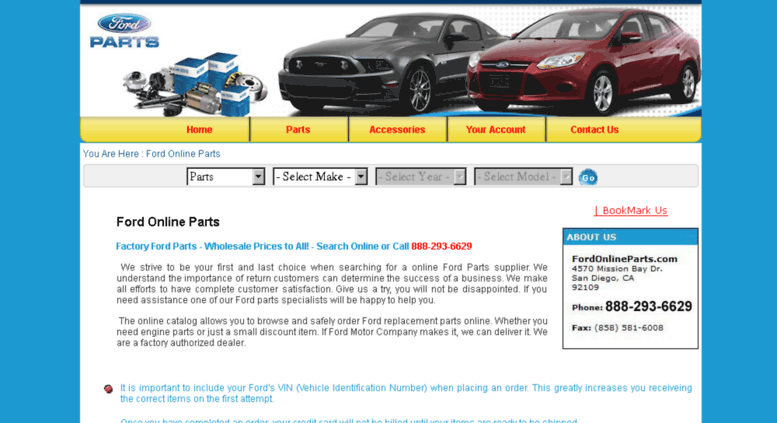This screenshot showcases a vintage design of the Ford Parts website. Prominently displayed at the top left is the iconic Ford logo accompanied by the word "Parts." Dominating the page is an image featuring two cars angled towards the right, juxtaposed with a pile of new parts and boxes positioned to their left. Beneath this image, a yellow bar spans the width of the page, featuring category names in red text: Home, Parts, Accessories, Your Account, and Contact Us. Centered below this bar, a series of drop-down boxes are displayed; the section header reads "You Are Here: Ford Online Parts." The first drop-down box has "Parts" selected, while the subsequent boxes, labeled Select Make, Select Year, and Select Model, remain unselected with the latter two grayed out. At the bottom left of the page, "Ford Online Parts" is reiterated, followed by a couple of paragraphs providing additional information. To the right of this text, there's a small "About Us" box. The rest of the page appears to be cropped out in the screenshot.